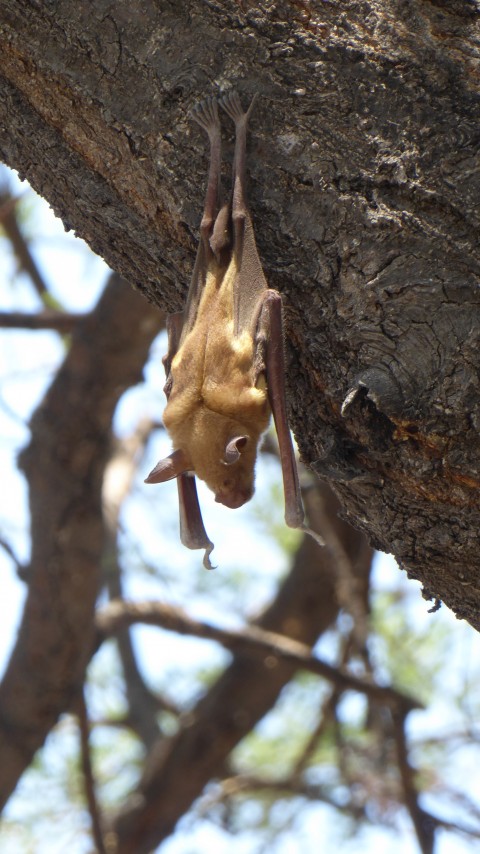In this detailed color photograph taken during the daytime, we see a small fruit bat hanging upside down from a large, diagonally oriented tree branch. The tree branch, which extends from the right side of the image to the top left, has a very rough, textured bark surface, and the bat's small, five-toed feet are securely latched onto it. The bat, which is light brown or beige in color, has fuzzy fur and rounded ears, with its wings neatly folded against its body. The bat is centered in the portrait-oriented frame, and its face is not visible from this vantage point. Surrounding the bat are blurred tree limbs and some green leaves, which are out of focus. A hint of light blue sky peeks through the foliage in the background, adding depth and context to the scene.